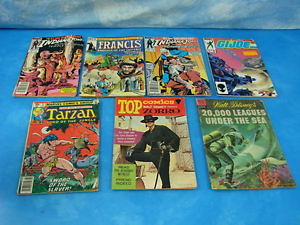The photograph, taken in color, is relatively small and depicts a collection of seven retro comic books spread out on an aqua blue surface, possibly a tarp or fabric. The background appears to be a similar light blue material with abstract white cloud-like patterns. Starting from the bottom left, there is a "Tarzan" comic, followed by a "Top Comics Zorro" featuring a black-masked man in a white-brimmed hat in the middle, and "20,000 Leagues Under the Sea" showcasing a large fish and a scuba diver to the right. On the top row from left to right, there is an "Indiana Jones" comic, a "Francis" comic, another "Indiana Jones" comic, and a "G.I. Joe" comic on the far right. The comic book covers are colorful and not preserved in protective bags, suggesting they are out for casual display.